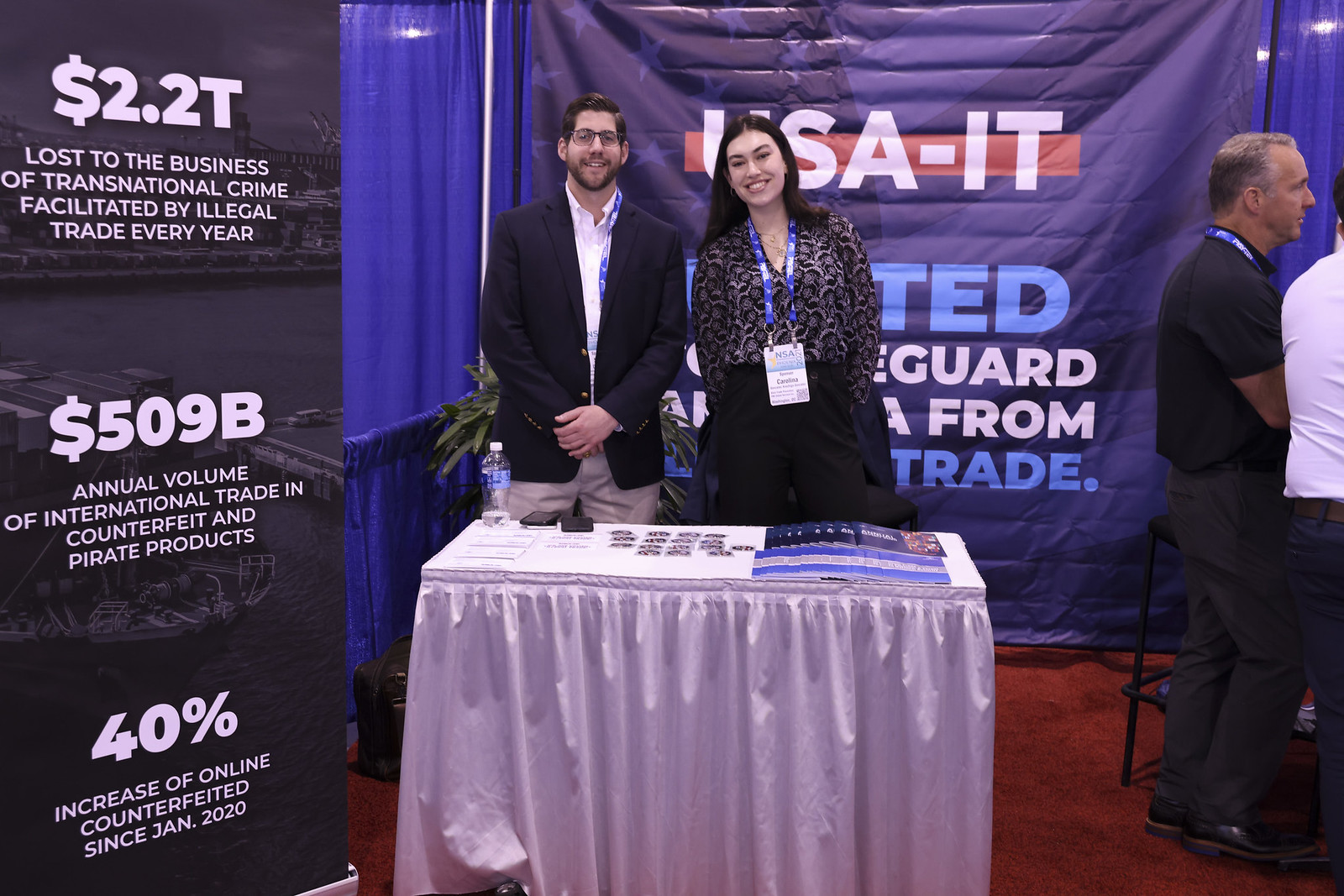This image captures a bustling scene at a conference, featuring a well-dressed man and woman standing behind a white satin-tipped table laden with various informational materials, including brochures, papers, and stickers. The man, a white gentleman with a mustache and beard, is attired in a dark suit coat with gold buttons, a white shirt, and khaki pants, and wears a blue and white lanyard partially concealed by his jacket. The woman beside him, identified by her badge as Carolina from NSA 2021, sports a black and gray leopard-print blouse, black pants, and gold necklaces. Both individuals are smiling and appear eager to engage with attendees.

Behind them, a banner prominently displaying "USA-IT" peaks out from behind Carolina’s head, while a green plant adds a touch of nature to the scene. To their left, a detailed sign lists staggering figures related to transnational crime: "2.2T lost to the business of transnational crime facilitated by illegal trade every year," "509 billion in annual volume of international trade in counterfeit and pirate products," and a "40% increase in online counterfeit since January 2020."

To the right, two additional conference attendees can be seen, one with short gray hair and another only partially visible. The setting is completed with a backdrop of blue curtains and red carpeted flooring, creating a professional and engaging environment dedicated to serious business discussions on combating financial crimes.